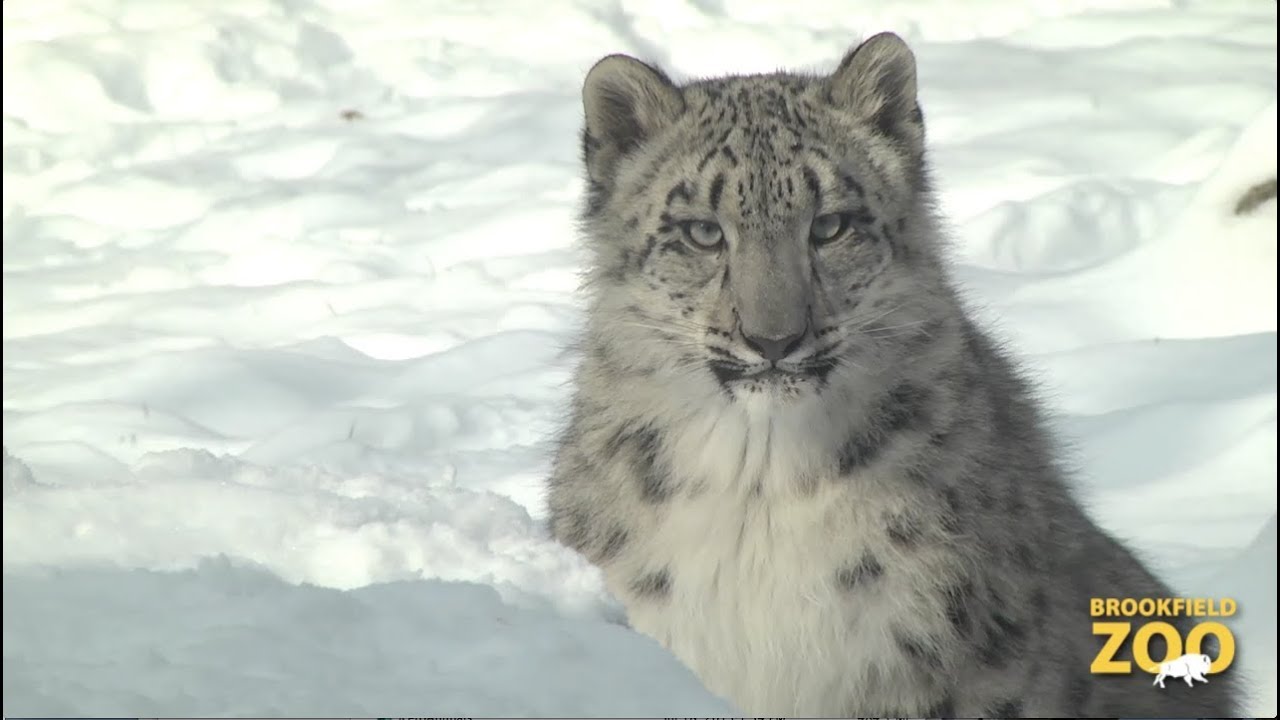This detailed photograph captures a magnificent wildcat, specifically a snow leopard, amidst a snowy landscape exclusively blanketed in white. The wildcat, with its lush, thick fur, showcases a muted pattern of black spots on a grey and white coat, which becomes more defined and detailed around its head, featuring darker black markings near the eyebrows and eyes. The cat's intense, almost silver or pale blue eyes are fixed straight at the camera with a piercing gaze. Its rounded ears and grey nose add to its distinctive appearance. The image is bathed in bright sunlight, reflecting off the surrounding snow and heightening the clarity of the scene. The depth of the snow is evident as it partially envelops the lower body of the animal. Notably, the bottom right corner of the photograph bears the text "Brookfield Zoo," further identifying the setting of this striking capture.